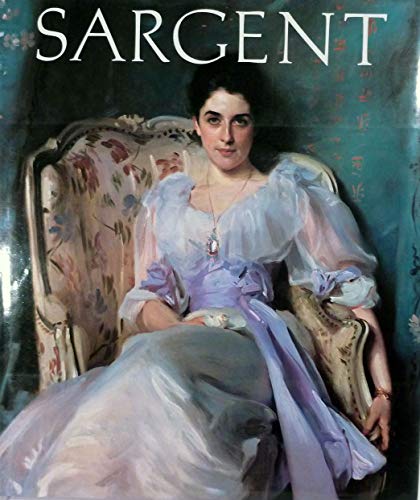This image appears to be an old oil painting of a Victorian-era woman seated in an ornate chair. The woman, who is white, features black hair swept up into a bun, black eyebrows, and red lips, exuding a stern yet composed demeanor as she faces the viewer. She wears a puffed-shoulder blue dress with accents of purple and white lace that has sleeves extending to her elbows. A notable accessory is her silver necklace with a white accent piece. 

The chair she occupies is richly detailed, described as white with a Victorian style, adorned with a floral pattern featuring red and blue flowers along with green leaves, and with an ornate gold-silver wooden design framing it. The woman is positioned sideways in the chair with her legs crossed, her left arm delicately wrapped around the side of the chair, and her right arm resting on her lap, holding an unseen object.

The backdrop is a light green or teal color, and the painting's upper section prominently features the word “Sargent” in large, white, uppercase letters. The entire composition exudes a sense of historic elegance and meticulous attention to the period's detail.